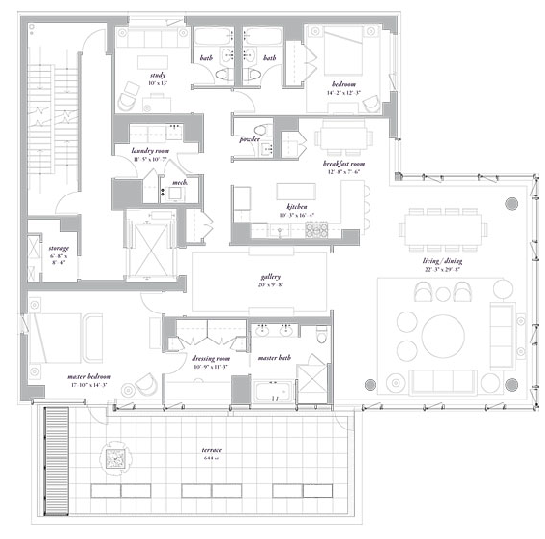This image depicts a detailed floor plan of a building, intricately divided into two distinct sections. The upper section resembles a large square area with an adjoining smaller square extension at its bottom edge. The lower section is a rectangular area that spans approximately half the length of the upper part. Notably, there are stairs located in the top left corner of the plan.

The floor plan, presented in black and gray shading, outlines various rooms and areas within the building, each clearly labeled with text. In some sections, tables are depicted, indicating functional spaces. For instance, there appears to be a designated dining area or a marketplace set up for selling goods.

One prominent area within the plan is a lounge, furnished with several chairs, a central table, and a couple of couches positioned around it, suggesting a space for relaxation or informal meetings. Additionally, a large meeting room is illustrated, featuring a substantial table surrounded by chairs, ideal for conferences or collaborative work.

In the bottom rectangular section, stairs are also indicated, ensuring connectivity between different building levels. The entire plan is organized into a grid pattern, which further aids in navigating the layout. While the schematic includes room labels and a basic layout, detailed furnishing is selectively shown, emphasizing areas like the lounge and meeting room while leaving other regions more abstract.